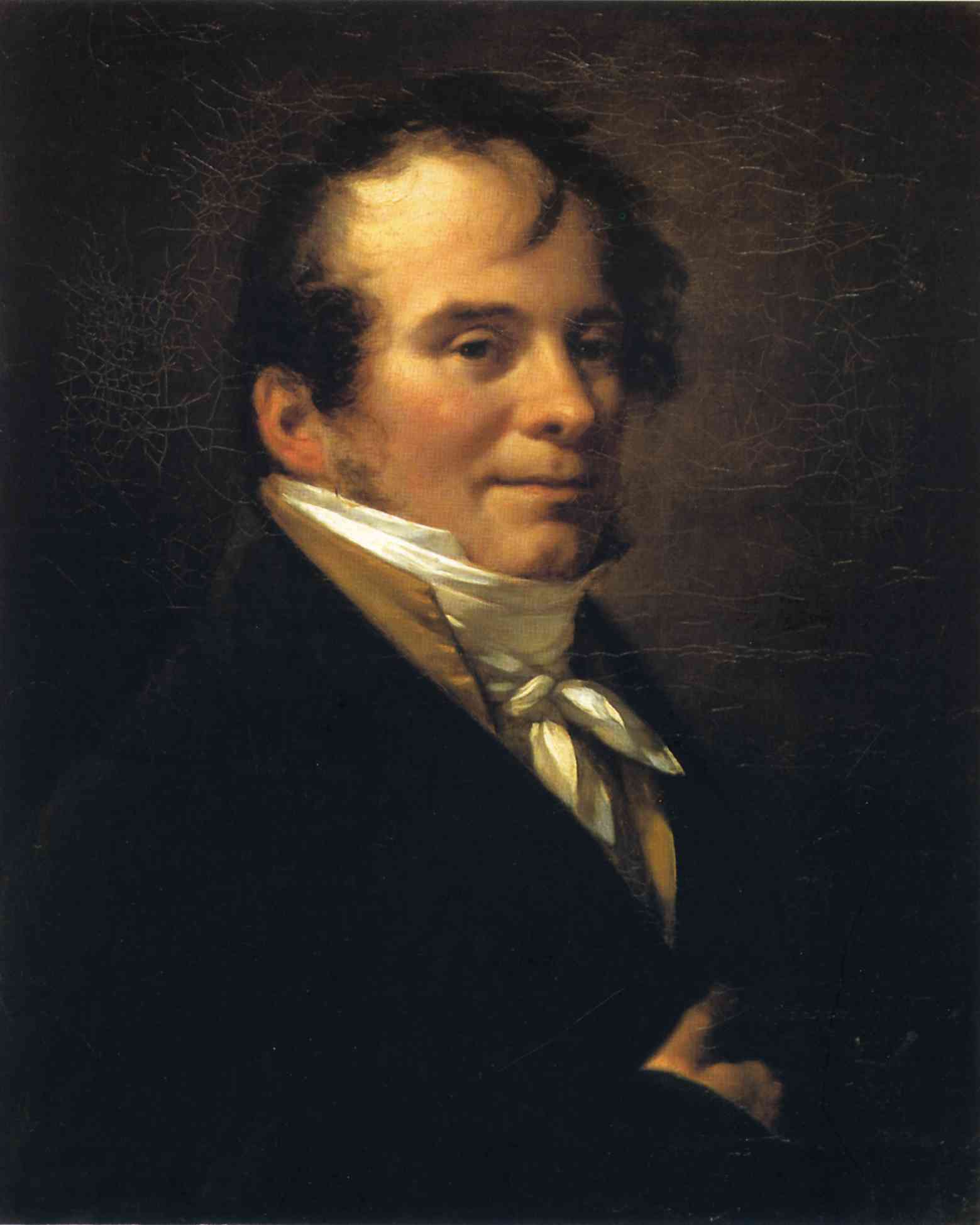This highly detailed portrait painting, titled "Monsieur Lavelle," by the artist Pierre Paul Proudhon, showcases a distinguished gentleman from the Victorian era. The painting, which is in portrait orientation, meticulously captures the likeness of a white man aged between 30 to 40 years with a slightly receding hairline and combed-over dark hair. He has long sideburns, a cleft chin, and a faint wisp of hair falling over his forehead. 

The man is dressed in a dark overcoat with a beige vest that features a stand-up collar. Around his neck, there is a layered white scarf tied in the style of an ascot with a knot in the front, giving it an elegant appearance. His right hand is tucked into his coat, striking a pose that exudes confidence and sophistication. 

The painting employs dramatic lighting, highlighting the man's face while keeping his shoulders and the majority of his body in darker shades. This creates a focal point on his detailed, realistic facial features. The dark background, with gradations of brown and beige, enhances the contrast and vintage feel of the artwork. The piece exhibits signs of age, with visible cracks suggesting it was created many hundreds of years ago, further emphasizing its historic and artistic value.